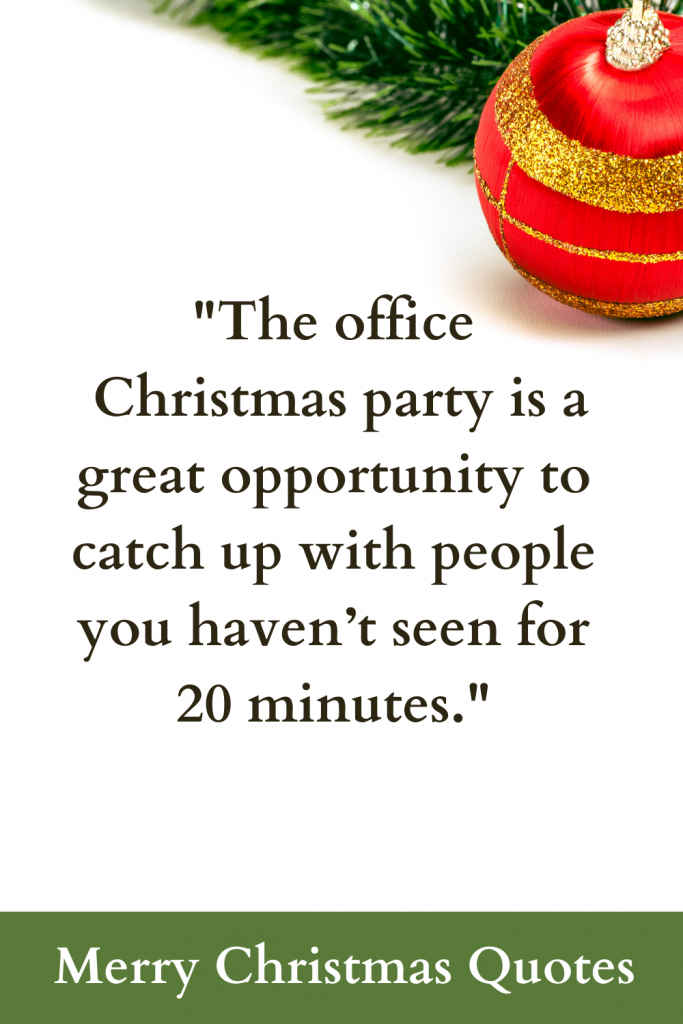This image captures a festive Christmas theme with several key elements. At the top right corner, a shiny red spherical ornament adorned with gold glitter bands—a thick stripe at the top, a thin stripe in the middle, and another thick stripe at the bottom—sits near spiky green branches of an evergreen tree. Centrally positioned against a white background in a serif font, a humorous quote reads, "The office Christmas party is a great opportunity to catch up with people you haven't seen for 20 minutes." At the bottom of the image, a light green banner runs across, featuring the text "Merry Christmas Quotes" in a white font. The overall color scheme includes festive shades of red, gold, green, white, and black, evoking a celebratory Christmas atmosphere suitable for a party or a Christmas card.